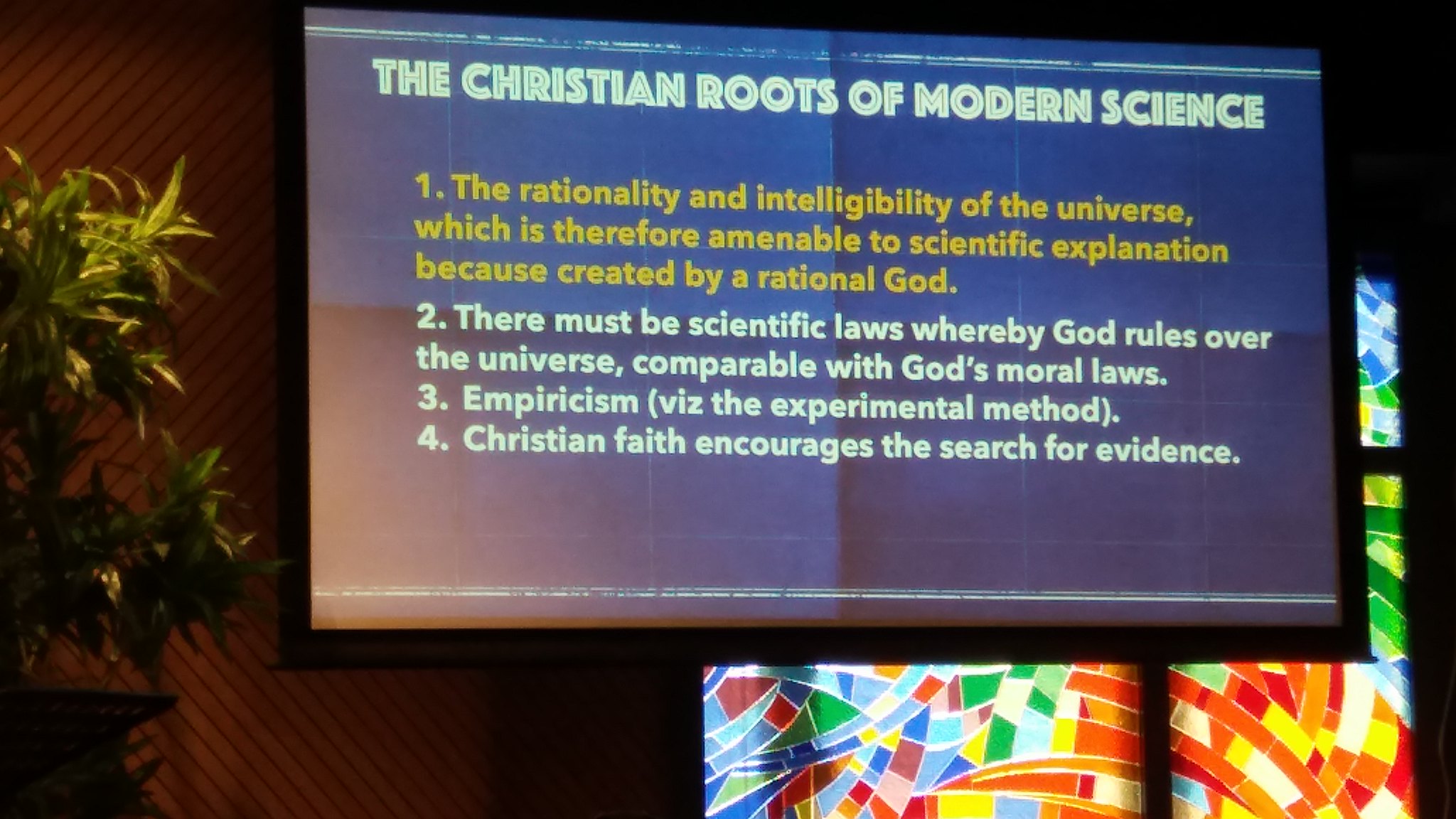The photograph captures a dimly lit church interior, where a prominent LCD screen or projector screen with a black border is displaying a PowerPoint presentation titled, "The Christian Roots of Modern Science," in all white uppercase letters. The slide features a blue and purple background with a numbered list of four points. The first point, highlighted in orange, states, "The rationality and intelligibility of the universe, which is therefore amenable to scientific explanation because created by a rational God." The subsequent points are in white text: "Two, there must be scientific laws whereby God rules over the universe, comparable with God's moral laws. Three, empiricism (viz. the experimental method). Four, Christian faith encourages the search for evidence." The left side of the image reveals a dimly lit plant or tree, while the background on the bottom right showcases a modern-looking stained glass window with vibrant colors, including red, white, blue, green, and yellow.